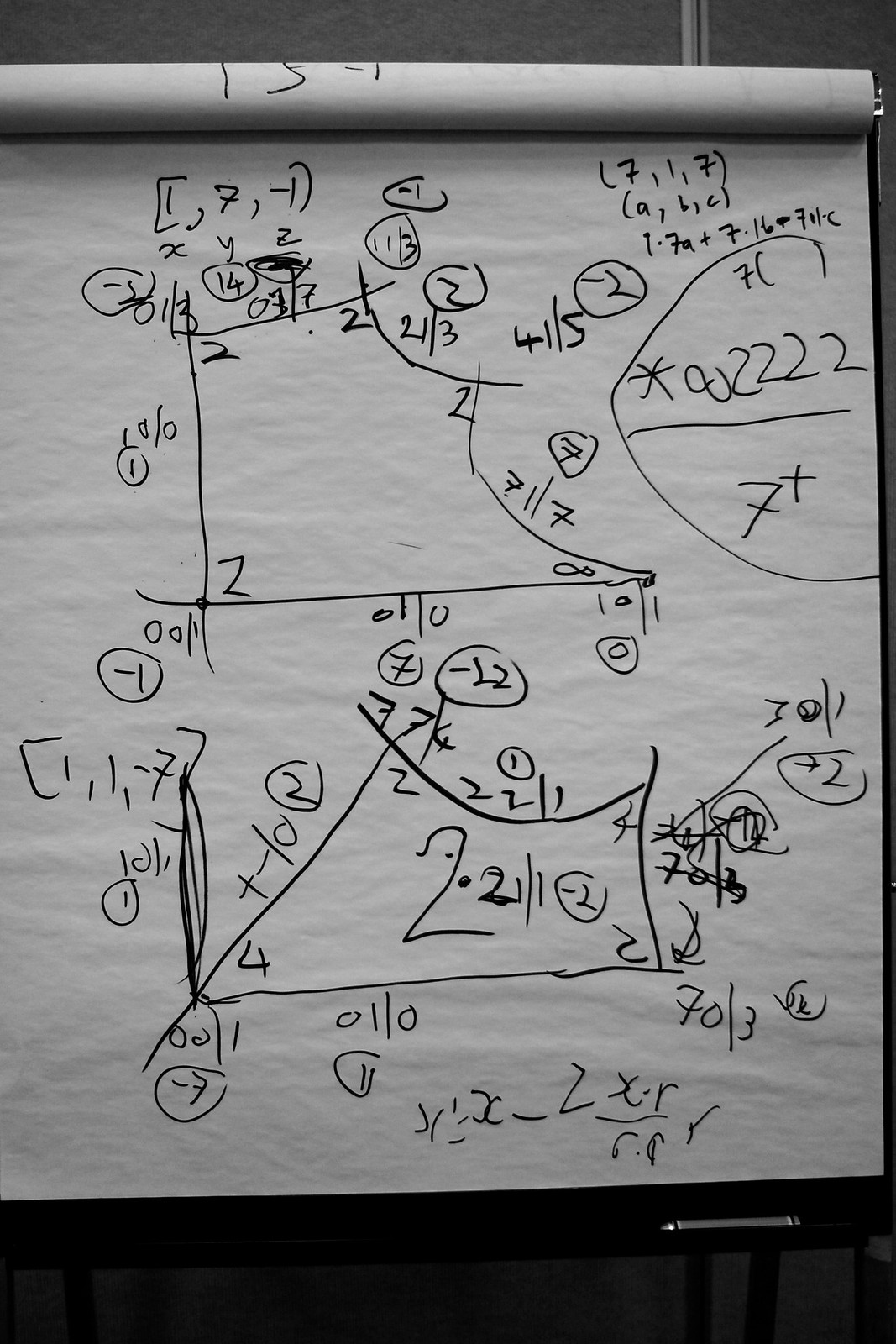This photograph features a large sheet of white paper adorned with various sketches and mathematical notations, likely produced in a classroom setting. The sheet, designed for use on a flip chart stand, has a visible curve at the top, indicating its readiness to be flipped over. At the bottom of the image, a black base with a silver support bar confirms its placement on a traditional flip chart stand.

The paper is filled with numerous black marker scribbles, indicative of a math or statistics class. Prominently displayed are vertical and horizontal lines, likely representing axes on a graph, with numerical values marked along these axes. On the right side of the sheet, there are parentheses containing different numbers, and below that, a hand-drawn bubble encapsulates another formula.

Additionally, the lower section of the paper features intersecting axes and more mathematical equations, further suggesting the instructional nature of the content. The entire composition reflects a dynamic classroom environment focused on complex mathematical or statistical concepts.